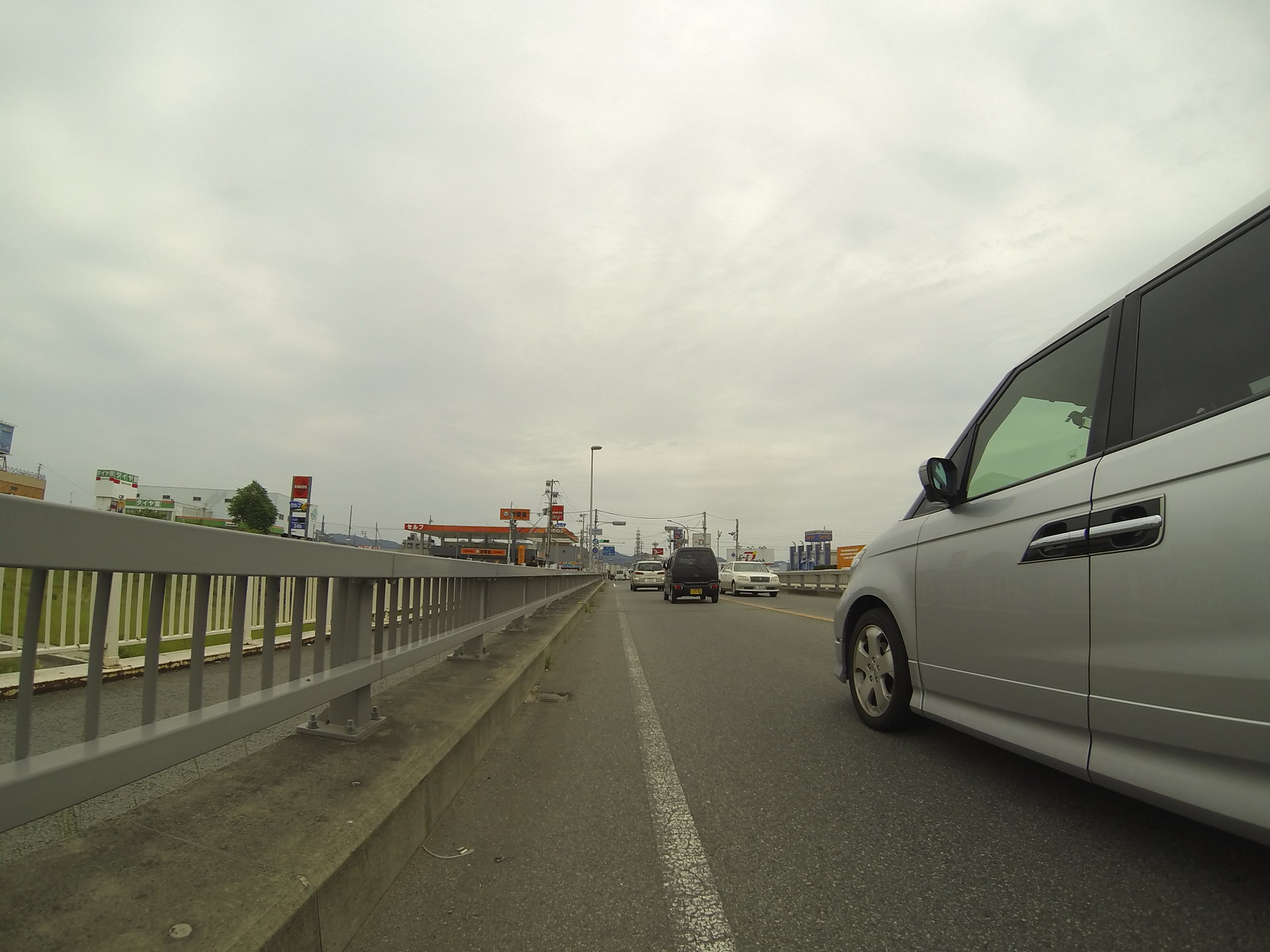Taken from the left side of the road, this photo captures the bustling scene of a bridge. The image likely snapped by someone on foot, shows traffic flowing in both directions. Vehicles travel on the left side, suggesting a country with left-hand driving. Among the cars, a silver hatchback stands out as the closest. Further down the road, a cluster of gas stations can be seen, adding to the urban ambiance. The perspective from the edge of the road offers a dynamic view of the bridge and the busy roadway.